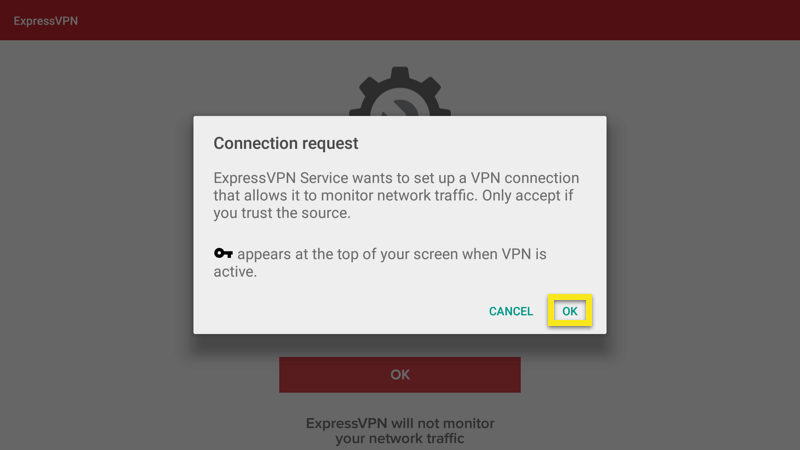"ExpressVPN Connection Request Notification: 

The ExpressVPN service is requesting permission to establish a VPN connection. This process involves setting up a secure tunnel that may allow the service to monitor network traffic for security purposes. The notification appears prominently at the top of your screen whenever the VPN is active. 

Options to respond include 'OK' to grant permission and 'Cancel' to deny the request. Please note that despite the initial wording, ExpressVPN assures users that their network traffic will not be monitored beyond the scope of ensuring secure and private browsing. Only proceed if you trust the source."